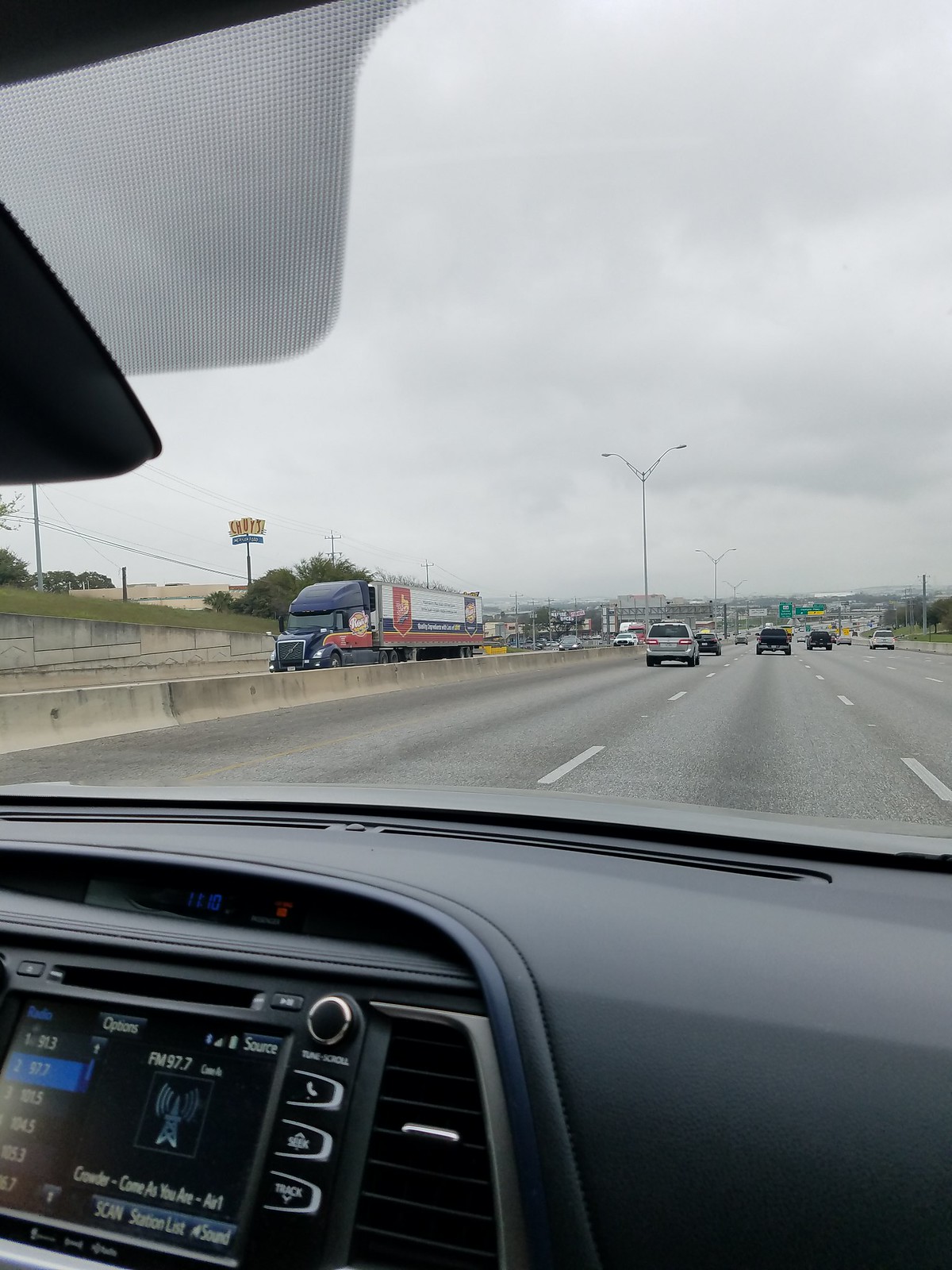This image, captured from the interior of a moving vehicle via a likely dashcam, offers a comprehensive view of the highway ahead. The car is traveling on a five-lane road with light traffic under an overcast sky filled with gray clouds, ensuring good visibility despite the weather. Green road signs hang above the lanes, though their text is not readable. Inside the car, the dashboard reveals controls for a radio station tuned to FM 97.7, playing "Come As You Are." The front view through the windshield shows multiple vehicles: a silver car in the passing lane, followed by a white car and two black cars ahead. On the opposite side, a massive truck with a black cab and white and red trailer is approaching, surrounded by other vehicles traveling in the opposite direction. A yellow sign with red lettering is visible to the left but unreadable. Additional details inside the car include a black dash, possibly hinting at a new model Toyota due to its in-dash info center, the visor down on the driver’s side, and various music control options displayed below the dashboard.